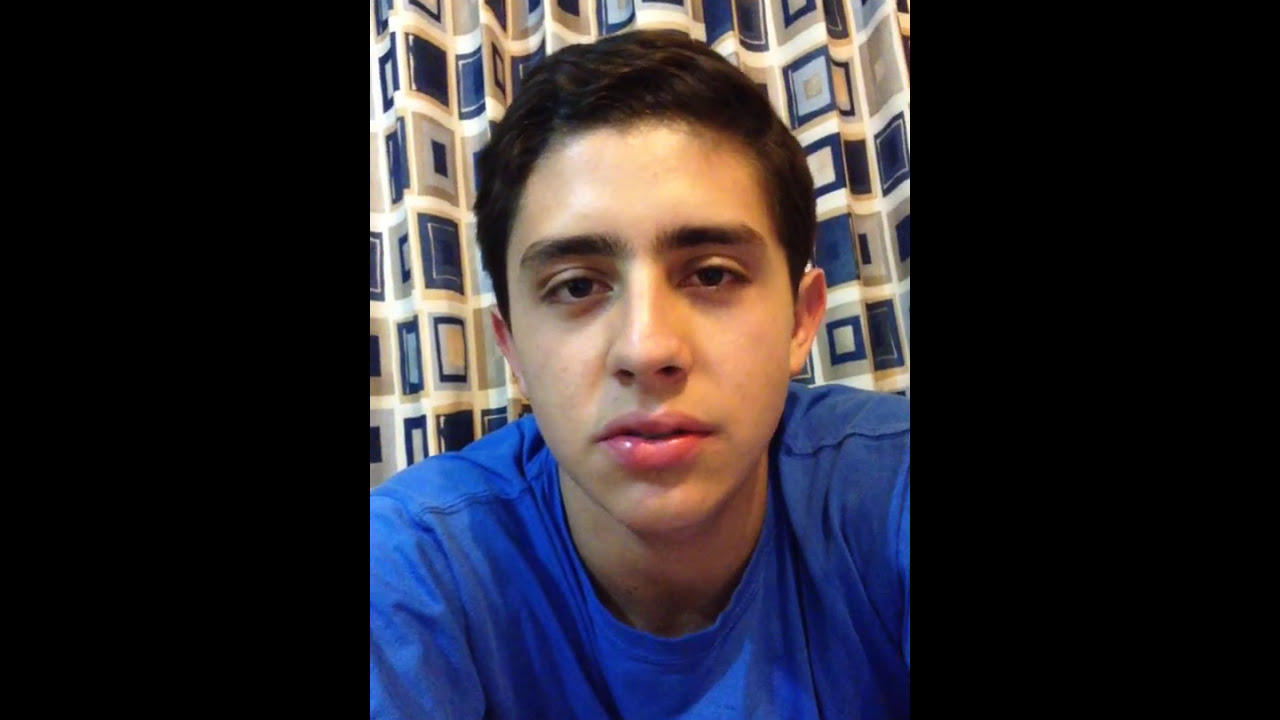In this color photograph, taken in portrait orientation, a young man is positioned directly in the center of the frame, from the shoulders up. He appears to be around 16 years old, with short black hair, olive-colored skin, and a blank, almost expressionless look on his face, as if he were talking into the camera. He is wearing a bright blue t-shirt. Behind him is a curtain that resembles a shower curtain or possibly just a regular curtain blocking a window. The curtain features a white background with various colored squares in shades of blue and beige. The setting appears to be indoors, likely in a bathroom. The lighting in the photo is good, casting a slight shine on the young man's forehead. The overall style of the image is realistic and photographic, capturing a candid selfie moment. There is no text visible anywhere in the image. The colors present include black, blue, tan, pink, brown, and yellow.